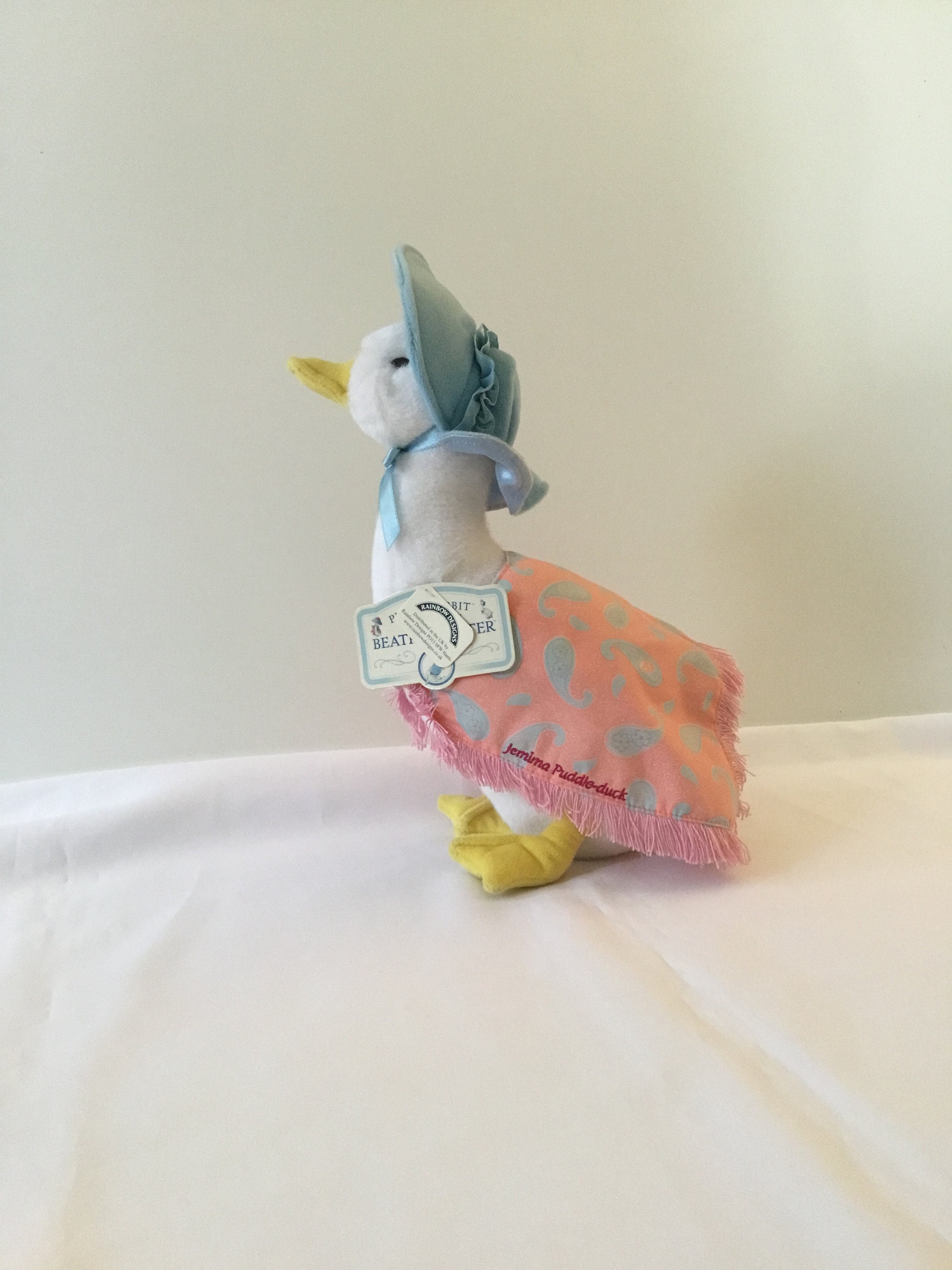This photograph depicts a small, white stuffed duck, reminiscent of characters from the Peter Rabbit series by Beatrix Potter. The duck is sitting upright on its own and is oriented towards the left. It has a yellow beak and yellow webbed feet. Adorning its head is a bluish-gray velvety bonnet, secured with a small blue ribbon. Across its back, the duck wears a pink shawl or blanket, with frayed edges resembling tassels. Embroidered in dark pink text on the shawl is the name "Jemima Puddle-Duck." Additionally, there is a product tag at the base of the neck. The scene appears to be set up for a resale listing, possibly for eBay, with the duck positioned on a white sheet and against a white background to emphasize its features and details.